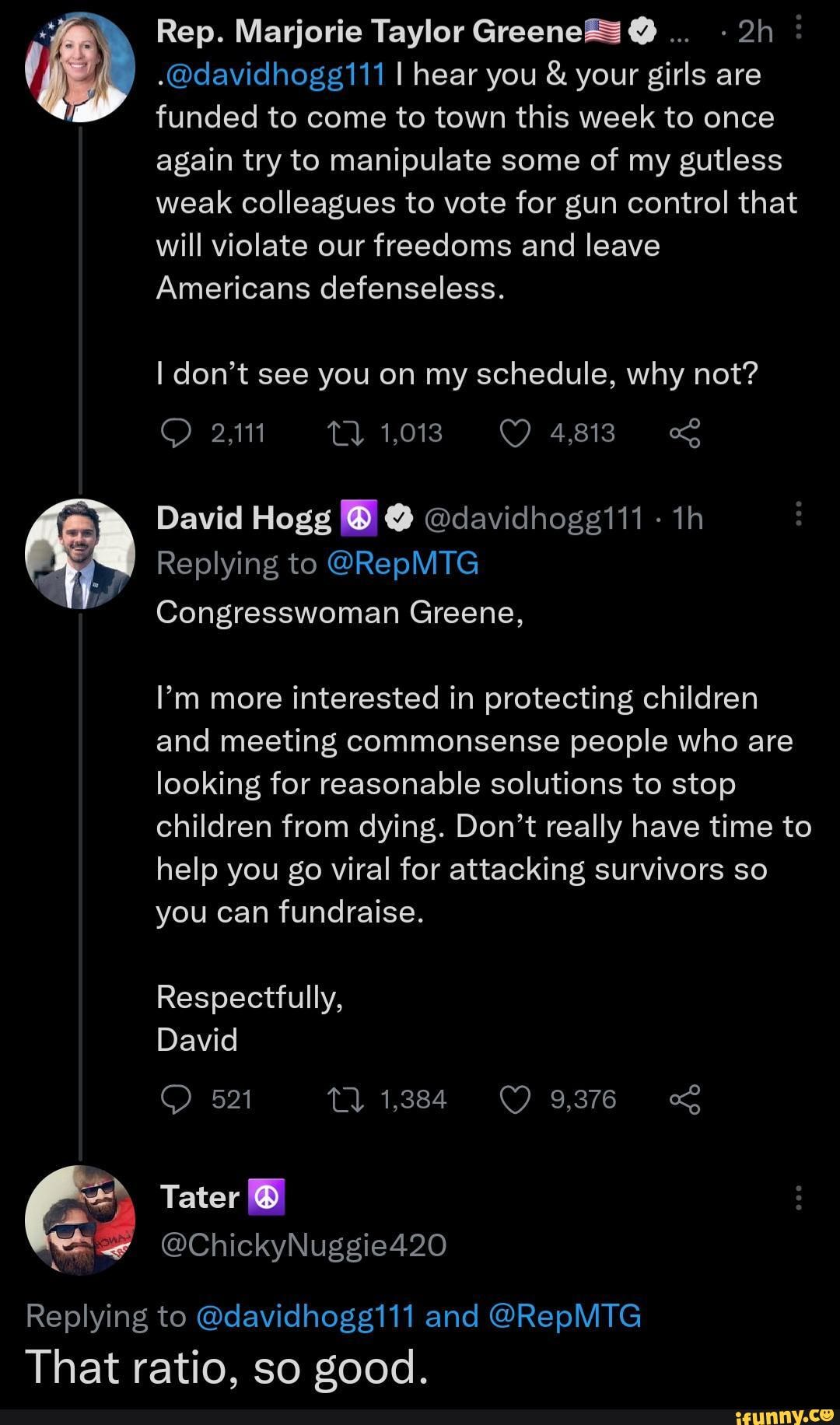The image depicts a Twitter exchange between Representative Marjorie Taylor Greene and gun control advocate David Hogg. 

In the first tweet, posted two hours ago, Rep. Marjorie Taylor Greene (@RepMTG) addresses David Hogg (@davidhogg111), stating, "I hear you and your girls are funded to come to town this week to once again try to manipulate some of my gutless weak colleagues to vote for gun control that will violate our freedom to leave Americans defenseless. I don't see you on my schedule, why not?" This tweet has garnered significant engagement with 2,111 comments, 1,013 shares, and 4,813 likes.

In response, David Hogg replied to Rep. Marjorie Taylor Greene, saying, "Congresswoman Greene, I'm more interested in protecting children and meeting common sense people who are looking for reasonable solutions to stop children from dying. I don't really have time to help you go viral for attacking survivors, so you can fundraise. Respectfully, David." Hogg's tweet has also received notable attention with 521 comments, 1,384 shares, and 9,376 likes.

Below this exchange, a user named Tater is also visible, although their interaction or comment is not specified in the provided description.